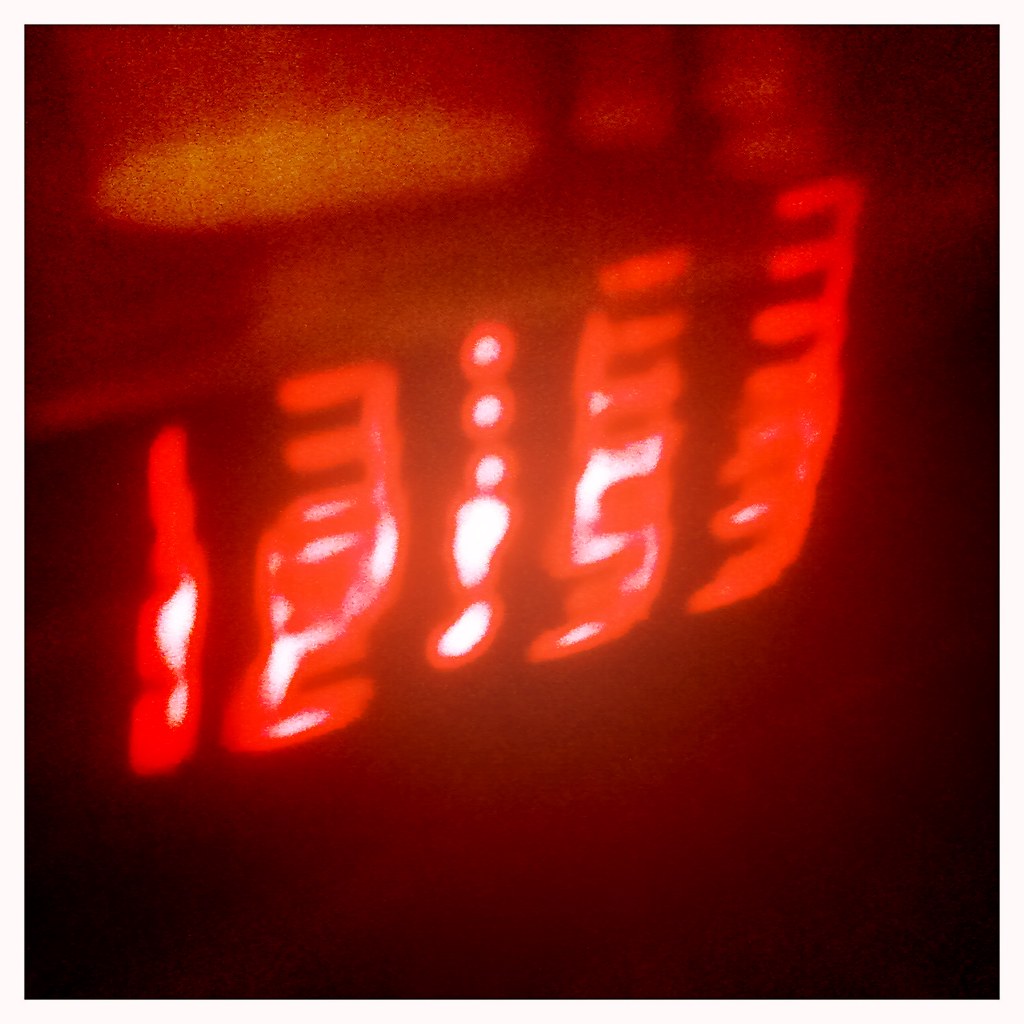The image is a square photograph with a predominantly dark background, especially concentrated around the bottom and side edges. The darkness fades into a slightly lighter dark red hue along the sides. The top portion of the image transitions to a bright, vivid orange color, drawing the eye upwards. 

At the center of the image, there's a neon light displaying blurred numbers, which appear to be reflected or doubled, creating a hazy effect. Despite the blurriness, certain numbers are distinguishable: a "1", a "3", followed by two indistinct characters, and another "3". This suggests the possibility of a digital clock, though it's unclear due to the image's lack of clarity. Additionally, there's a white number resembling a "5" along with some scattered white dots in the vicinity of the light. The central light, surrounded by these numbers and dots, shines a bright orange, standing out starkly against the darker backdrop.